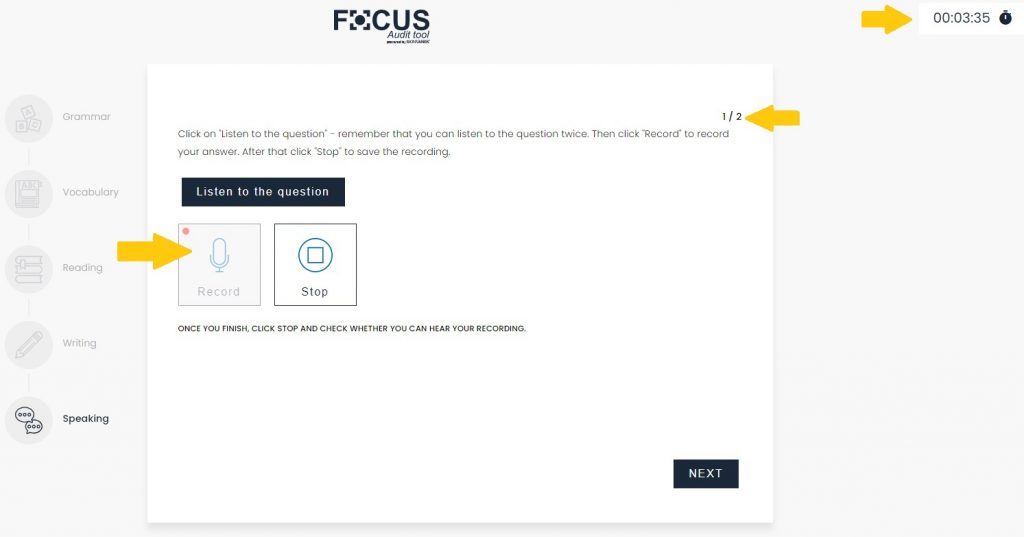This screenshot appears to be from a web application featuring an audit tool. The background at the top is gray, with the title "FOCUS" prominently displayed in the center using a black font. The "O" is stylized within a squared shape, adding a unique design element to the title. Below the title, in a smaller font, it reads "audit tool."

In the upper right corner of the screen, there is a yellow arrow pointing towards a white square that displays a timer reading "00:03:35" in black font, accompanied by a small black bomb icon.

Further down, there is a white rectangular area marked at the top with "1/2" and another yellow arrow pointing to this designation. The instructions read, "Click on the listen to question. Remember that you can listen to the question twice. Then click record to record your answer. After that, click stop to save the recording."

Beneath these instructions is a black rectangle with white text stating "Listen to the question." Below this, there are two squares. The first square highlights "Record" with a blue microphone icon in the center, emphasized by another yellow arrow pointing directly at it.